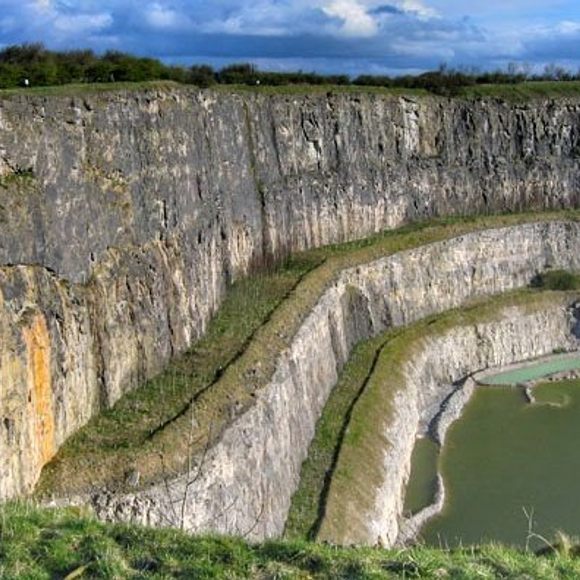This color photograph captures an outdoor scene of a limestone quarry with a series of large, stone steps forming its walls. The steps, characterized by their light gray, tan, and dark gray hues, ascend from right to left, with the tallest on the far left. The tops of these steps are blanketed with green vegetation, possibly grass or moss. Above this, the background features a line of trees or shrubs. At the bottom of the image, there's a close-up view of grass with sparse, leafless shrubs or twigs, indicating seasonal dormancy or death. The quarry's base on the bottom right is partially flooded, with stagnant greenish water. Dominating the background, a dramatic blue sky filled with dark blue and white clouds hovers above, adding a sense of impending weather.